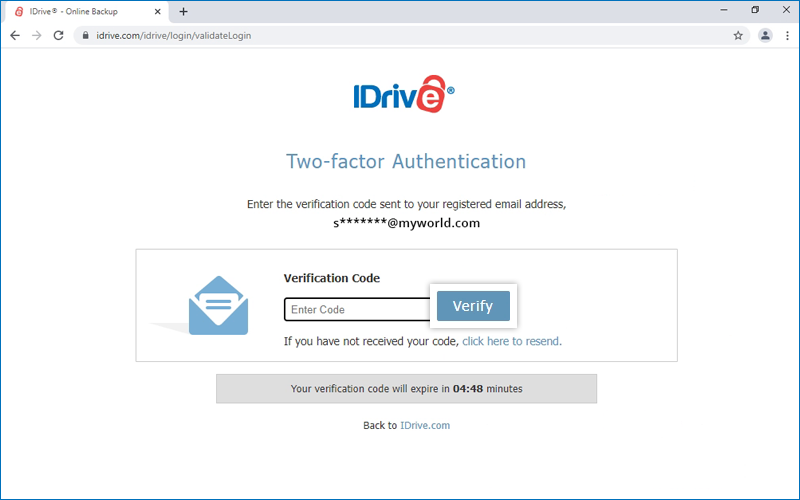The image showcases a section of the iDrive.com website, specifically a two-factor authentication page. Dominating the center of the web page is the iDrive logo, featuring the text "iDrive" in blue, with a white 'E' overlaid by an orange-red padlock icon, symbolizing security. Beneath the logo, bold blue text reads, "2-factor authentication." The instructions "Enter your verification code, sent to your registered email address," are followed by a partially obscured example email "S*****@myworld.com," hinting at the user's obscured email address for privacy. Below this, an input box is provided for the user to enter the verification code. Adjacent to the input box on the right is a light blue button with the word "Verify" written in white, inviting the user to confirm their identity.